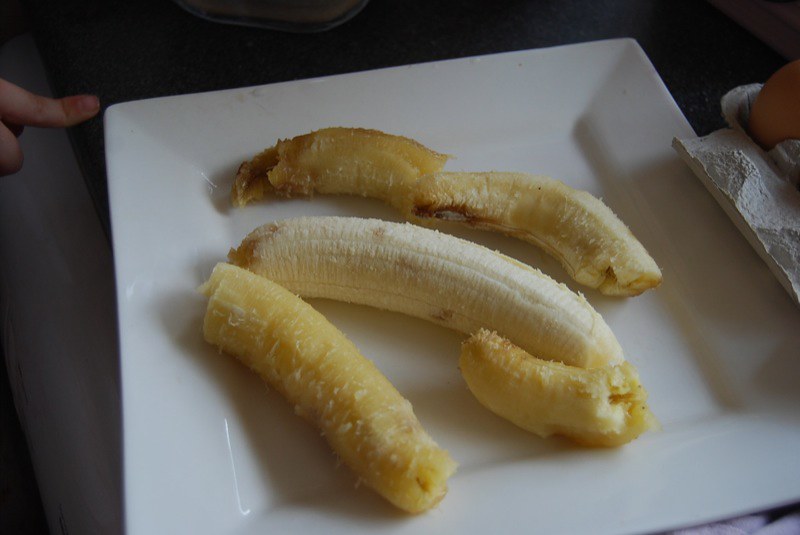In the image, a plain white plate holds a variety of bananas. Positioned prominently is a fresh, regular banana with visible bruising and a slightly overripe top. Surrounding the fresh banana are four pieces of fried bananas, markedly different in quality.

Two of the fried bananas appear perfectly cooked, showcasing a deep yellow hue with a texture that suggests a coconut-like crispiness, although it might just be the natural frying process. They retain their shape well and look appetizing.

In stark contrast, the other two fried bananas seem less appealing. One is notably thin and over-fried, having turned into a crunchy, brown-black remnant with hardly any banana inside. The other problematic piece is collapsed into a curve, suggesting insufficient banana content for proper frying. It is marred by black-brown patches, indicating uneven cooking.

A person's finger is also visible in the background, around the edge of the plate, adding a sense of scale to the image.